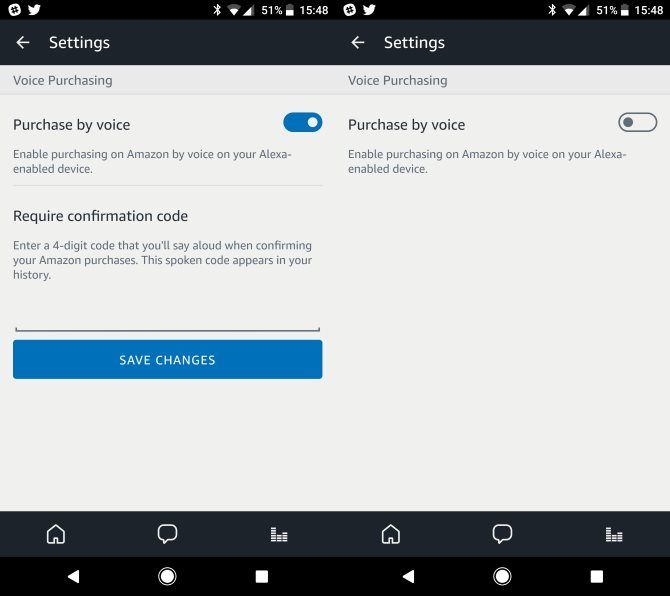This image displays a screen within an app, specifically focusing on voice purchasing settings. The photo is almost square and shows two sections side-by-side, likely for comparison purposes. 

**Top Bar:**
- The top of the image features a thin horizontal black bar containing several icons:
  - A sideways pound sign inside a white circle on the far left
  - Twitter icon in white
  - Bluetooth icon
  - Wi-Fi and cellular signal meter
  - Battery icon indicating 51% charge with a white meter halfway up the vertical battery
  - Time displayed as 15:48

**Left Section:**
- Beneath the top bar, this section displays voice purchasing settings:
  - The heading "Voice Purchasing"
  - Sub-heading "Purchased by Voice" in black font
  - A slider toggle that is positioned to "On"
- Below this, there is a thin border line followed by:
  - A prompt "Require Confirmation Code" 
  - An input field represented by a bracket with an underscore where a code can be typed
  - A "Save Changes" button

**Right Section:**
- Mirroring the layout of the left section but with slight differences:
  - Shows "Voice Purchasing"
  - "Purchased by Voice" text, similar to the left, but the slider toggle is positioned to "Off"
- There are no further options or input fields displayed below this section, in contrast to the left side.

**General Description:**
- The image aims to compare the settings for voice purchasing when "Purchased by Voice" is toggled on versus off. The left part shows the settings options when the feature is enabled, while the right part shows the interface when it is disabled. The lack of a defined border between the two sections suggests a seamless comparison within the app’s settings page.